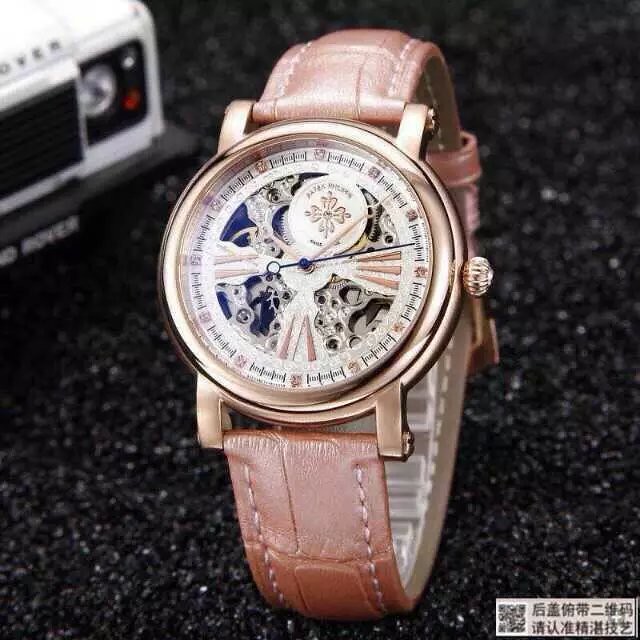This color photograph showcases a luxurious Patek Philippe wristwatch with a detailed view emphasizing the intricate craftsmanship. The watch features an embossed brown leather strap and a distinctive round brass covering that attaches the strap to the circular face. The face of the watch is gold, adorned with Roman numerals at the three, six, and nine o'clock positions, highlighted by a small pink gemstone where the hours would be marked. The black second hand and gold hour hand point to approximately 1:13. The dial has a clear face, revealing the exquisite silver and gold gears within, while a round logo between the twelve and one reads "Patek Philippe Geneva." On the lower left of the image, Asian characters and a QR code are present. 

The watch is set against a dark, almost blacktop-like background. To the left of the watch, partially in view, is a white toy Range Rover with a black front bumper, black grille, and red and clear crystal lights, adding a compelling juxtaposition to the elegant timepiece. The word "Rover" can be seen clearly on both the hood and bumper of the miniature vehicle. In the backdrop, a cluster of black, coal-like crunched rocks is visible, subtly enhancing the texture and depth of the image.